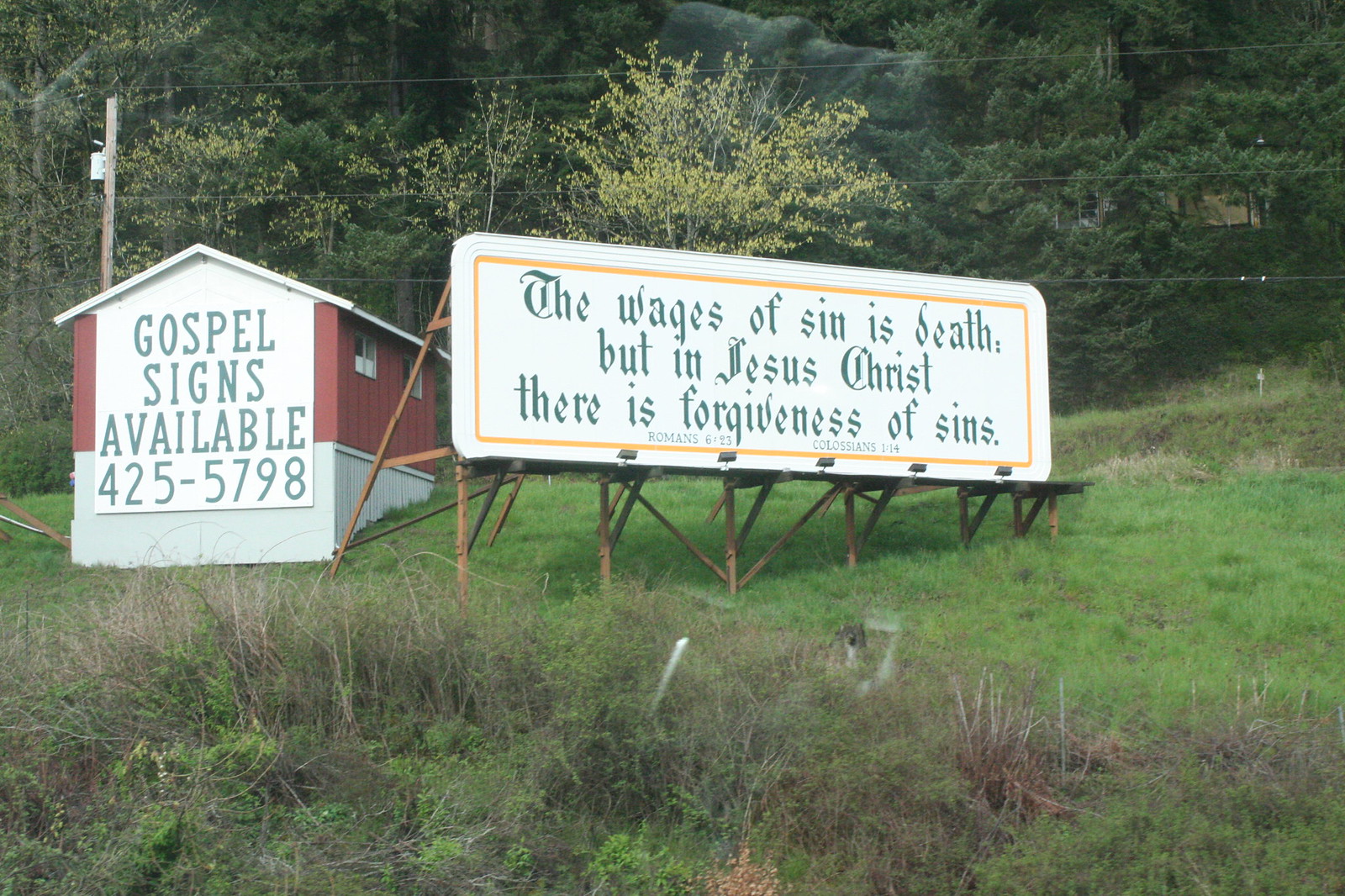In this roadside scene, you observe a picturesque green hill, its slopes covered with lush grass and dense brush at the base. Standing prominently on this hill is a wooden sign, supported by several sturdy posts beneath and a rear post ensuring its upright position. 

The sign itself is horizontally rectangular and painted white, bordered elegantly with a rich gold trim. It features a message written in an ornate, old-style cursive font: "The wages of sin is death, but in Jesus Christ there is forgiveness of sins." Below this, in more modern typed lettering, is a citation of a Bible verse.

Adjacent to this evocative sign, to the left, stands a quaint, small building with striking red walls and a gable roof, clad in siding. This building bears its own sign, informing passersby that "Gospel signs available" accompanied by a phone number for further inquiries.